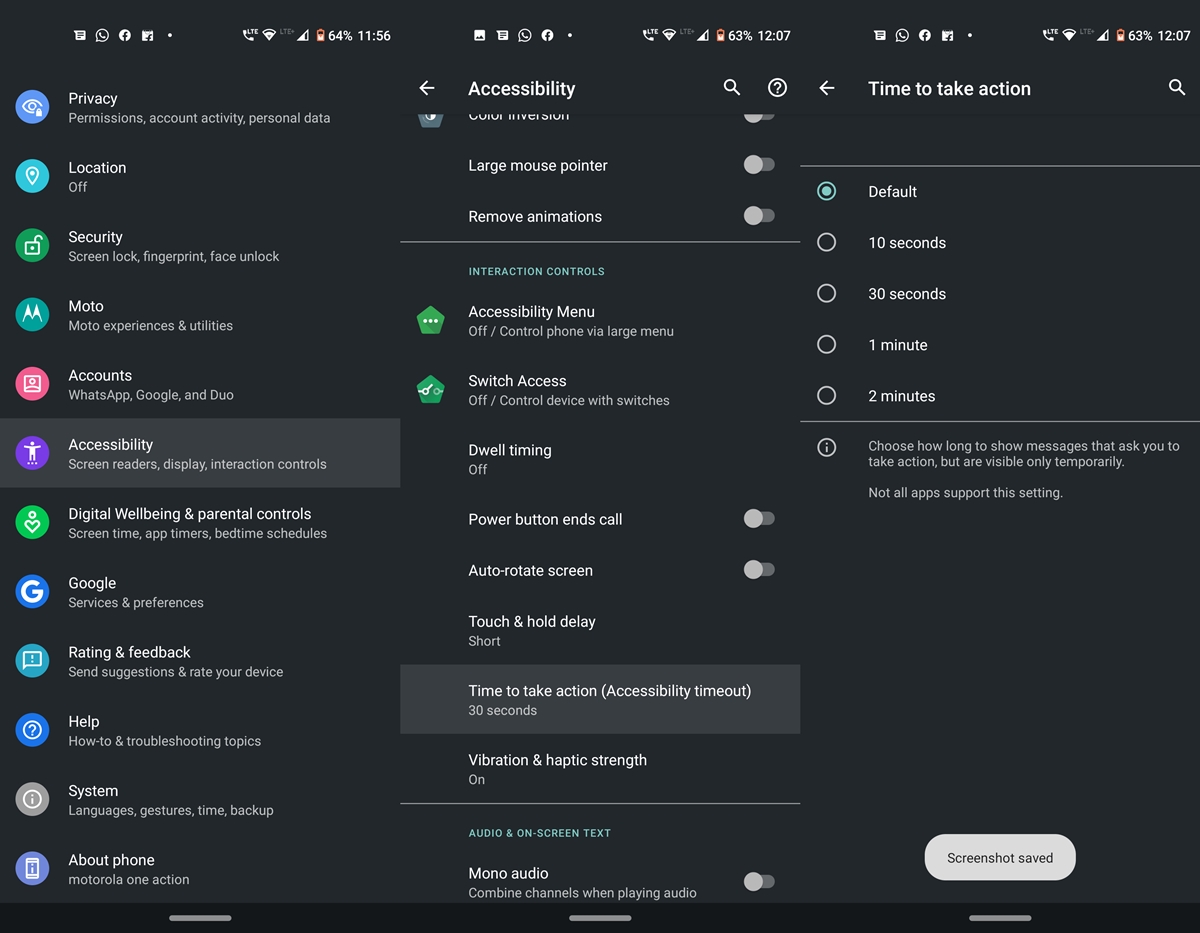The image displays a detailed triptych of phone screenshots arranged side-by-side, illustrating various settings and menus. 

### Left Screenshot:
- **Top Row Icons**: Instagram, WhatsApp, Facebook, and another application.
- **Right Side Elements**: Phone signal, Wi-Fi signal, battery at 64%, and the time displayed as 11:56.
- **Content**: A list of menu items in black-and-white text:
  - Privacy
  - Location
  - Security
  - Accounts
  - Accessibility (highlighted in gray)
  - Digital Well-being
  - Parental controls
  - Google
  - Rating and Feedback
  - Help
  - System
  - Phone 

### Middle Screenshot:
- **Header**: A back arrow pointing left with the title "Accessibility."
- **Dropdown Items**: Though the first item is not visible, the subsequent list includes:
  - Large Mouse Pointer
  - Remove Animations
  - Interactive Controls
  - Accessibility Menu
  - Switch Access
  - Dwell Timing
  - Power Button and Call
  - Auto-Rotate Screen
  - Touch and Hold
  - Time to Take Action (highlighted in gray)
  - Accessibility Timeout
  - Vibrate and Haptic Feedback Strength
  - Audio and On-Screen Text
  - Mono Audio
- **Right Side Elements**: Phone signal, Wi-Fi signal, battery at 63%, and the time displayed as 12:07.

### Right Screenshot:
- **Top Elements**: Same technical details as the left:
  - Phone signal, Wi-Fi signal, battery at 63%, and the time displayed as 12:07.
- **Header**: Shows an arrow pointing left labeled "Time to Take Action," indicating a form of navigation within the accessibility settings.
- **Options**: Settings for "Time to Take Action" with selectable timers:
  - Default (set to "On")
  - 10 Seconds
  - 30 Seconds
  - 1 Minute
  - 2 Minutes

### Bottom Notification:
- A small white bubble with gray text reads "Screenshot saved," indicating a recent screen capture.

This descriptive caption effectively communicates the contents of the image and the intricate details in each screenshot.